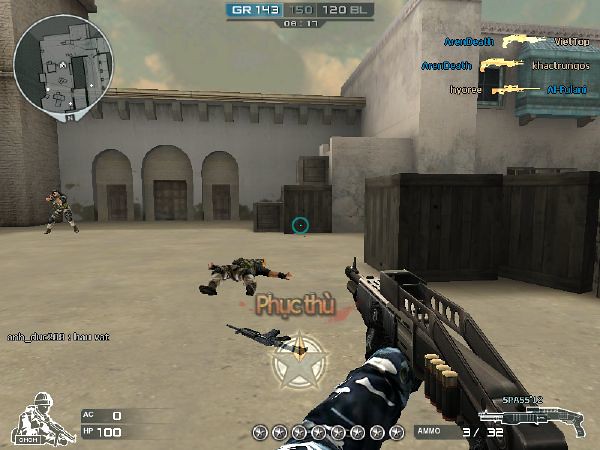In this screenshot from a first-person shooter video game, the player views the action from their avatar's perspective, vividly capturing a high-stakes moment. The player's left hand firmly grips a large, brown firearm while wearing a blue and black camouflage sleeve, emphasizing their readiness for combat. Displayed at the bottom of the screen is an icon of the gun in use, detailed ammunition statistics, and a score accompanied by a soldier icon.

In the upper right corner, additional gun icons and player usernames provide a quick reference to the team dynamics. The upper left corner features a compact map portion within a circular frame, offering a strategic overview of the surroundings.

The scene is set in a gray and tan compound, likely part of an exterior building complex. At the foreground, a character is sprawled on the ground, adding to the intensity and urgency of the environment. This detailed and immersive depiction highlights the intricate design and interactive elements that define the gaming experience.